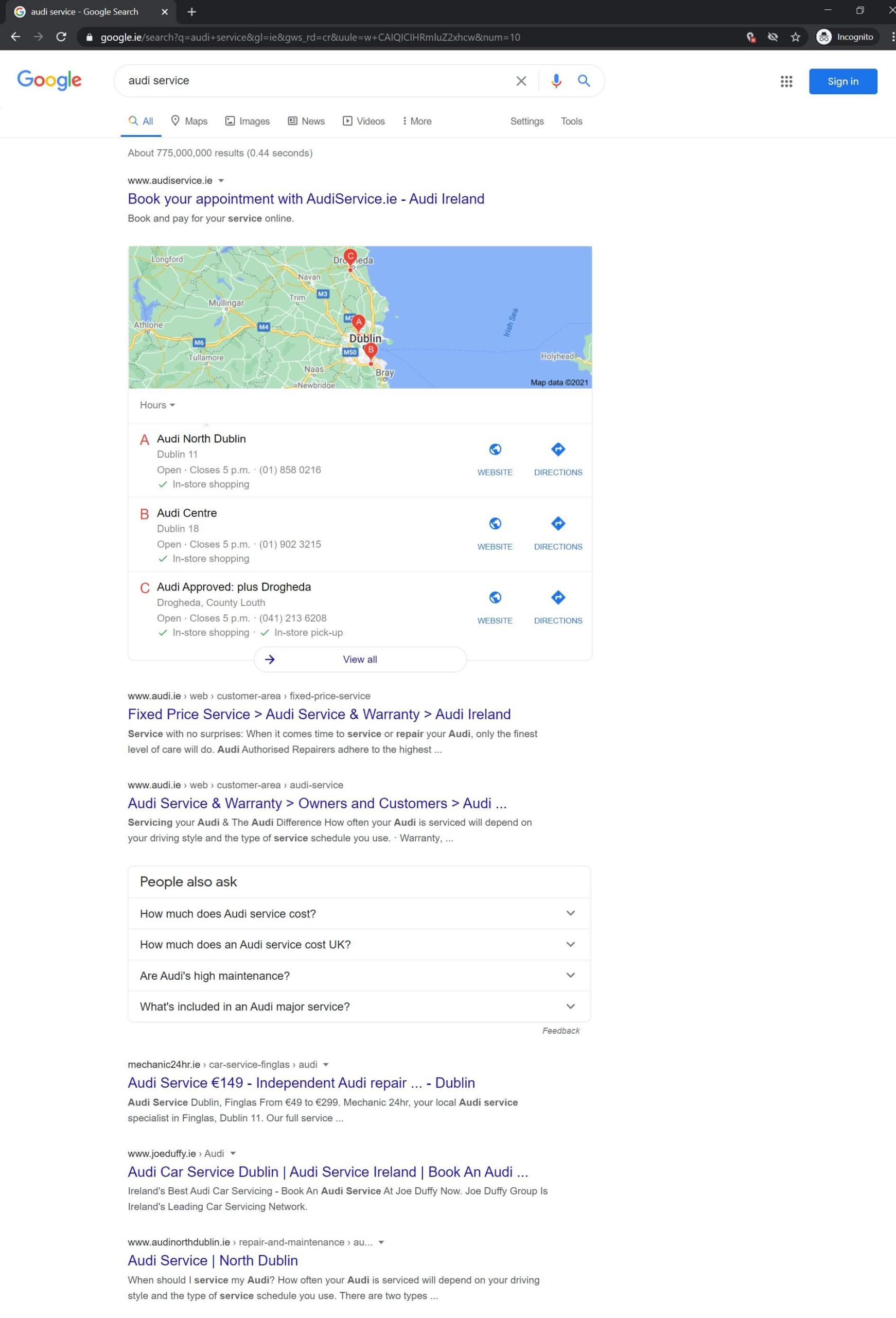The image depicts a Google search result page for the query "Audi Service." The search menu shows the 'All' tab selected. At the top of the page, there is a map centered over Ireland with three marked locations, labeled A, B, and C. These markers represent three Audi service centers: Audi North Dublin, Audi Coot Centre, and Audi Approved Plus Drogheda. Each of these listings includes website links and directions.

Below the map, there are additional search results with titles such as "Fixed Price Service," "Audi Service and Warranty," and "Audi Ireland," each accompanied by brief descriptions. This detailed layout provides various options for users seeking Audi services and information in Ireland.